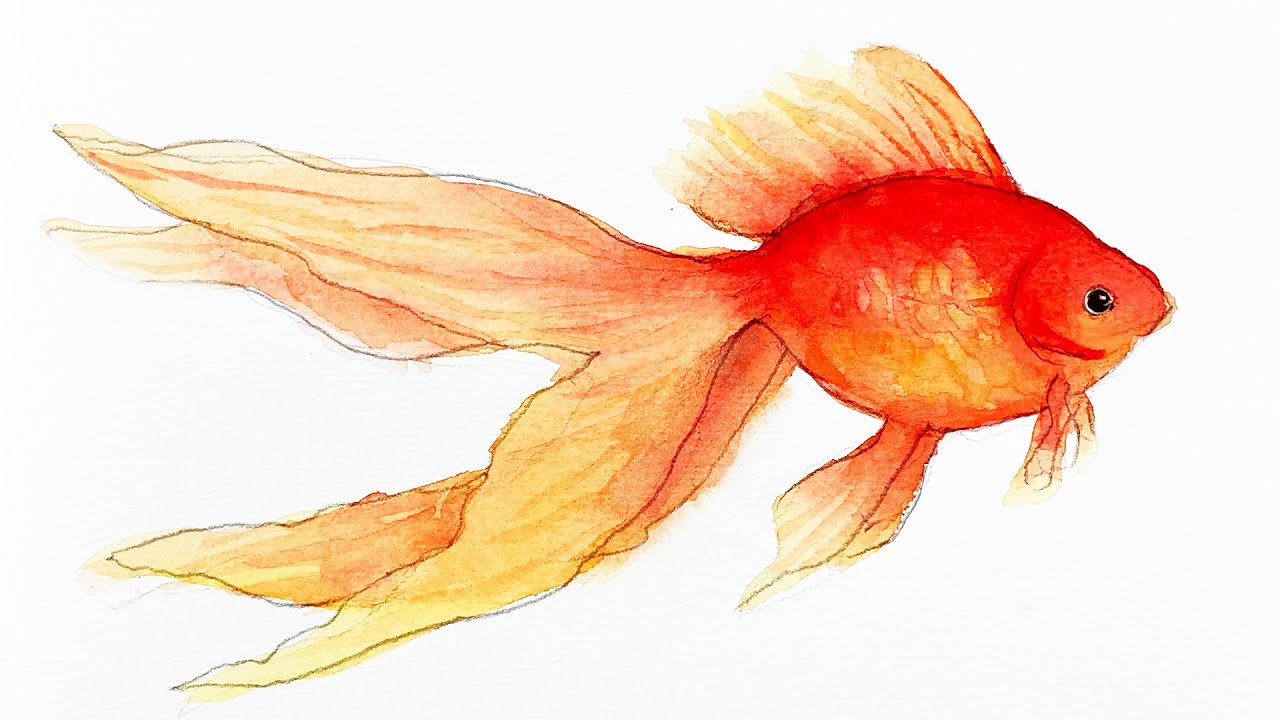This image portrays a meticulously detailed watercolor painting of a plump goldfish with a distinctively oval body. The fish features small, delicate fins beneath its head and a prominent dorsal fin. Its most striking attribute is its tail, formed by two sets of long, wavy fins, giving the impression of four distinct prongs, which extend beyond the length of its body, reminiscent of an angelfish. The fish's coloration is a vibrant gradient; its top is a bright orange-red, transitioning to yellows and oranges on the underbelly, with touches of pink. The fins are a light pink, accented with red outlines. The fish has striking black pupils, set against the primarily orange and yellow hues. This artistic representation, which could be interpreted as a blend of a sketch and a painting, is set against a plain white background.